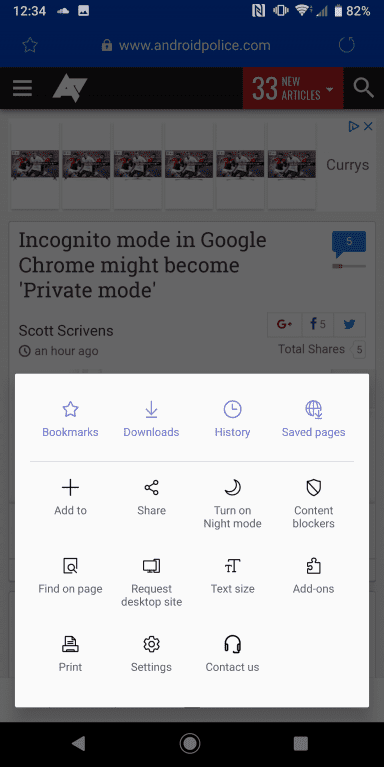This screenshot captures a detailed view of a mobile browser interface on www.androidpolice.com, prominently featuring a pop-up menu. At the top of the screen, we see typical mobile status indicators: the time "12:34," a cloud icon, and a photo icon depicting mountains, followed by a logo resembling an "N" or possibly a watch symbol. To the right, a phone icon with vibrating arrows, a Wi-Fi symbol, and a signal strength meter showing one bar are displayed. The battery icon, almost full at 82%, is positioned next to this.

Below these indicators, the URL bar contains several elements: a solid blue background unstarred favorite icon, a secure lock icon, the URL "www.androidpolice.com," a refresh button, and a menu icon represented by three vertical lines. The website's logo, a combination of upward and downward-facing triangles along a diagonal line, is also visible. Next to the logo, a red notification box displaying "33 new articles" alongside a dropdown arrow is present, complemented by a search bar.

The central portion features an advertisement from Curry's, delineated into six panels, each showing a grayscale image of individuals playing soccer. The main article headline reads "Incognito mode in Google Chrome might become private mode," with information showing five comments and a publication time of an hour ago by Scott Scrivens. Sharing options include Google+, Facebook, and Twitter, with a total of five shares.

Currently open is a detailed menu of browser actions, organized into four rows by four columns. The first row displays options for Bookmarks, Downloads, History, and Saved Pages, all highlighted in a bluish-purple font with respective icons. A thin gray line separates this from the second row, containing the options Add to, Share, Turn on Night Mode, and Content Blockers, each with corresponding icons. The third row offers Find on Page, Request Desktop Site, Text Size, and Add-ons, also paired with icons. The final row lists Print, Settings, and Contact Us, with the fourth cell left empty.

At the very bottom of the screenshot, a black rectangular control bar features a play button, a record button, and a stop button, all rendered in gray.